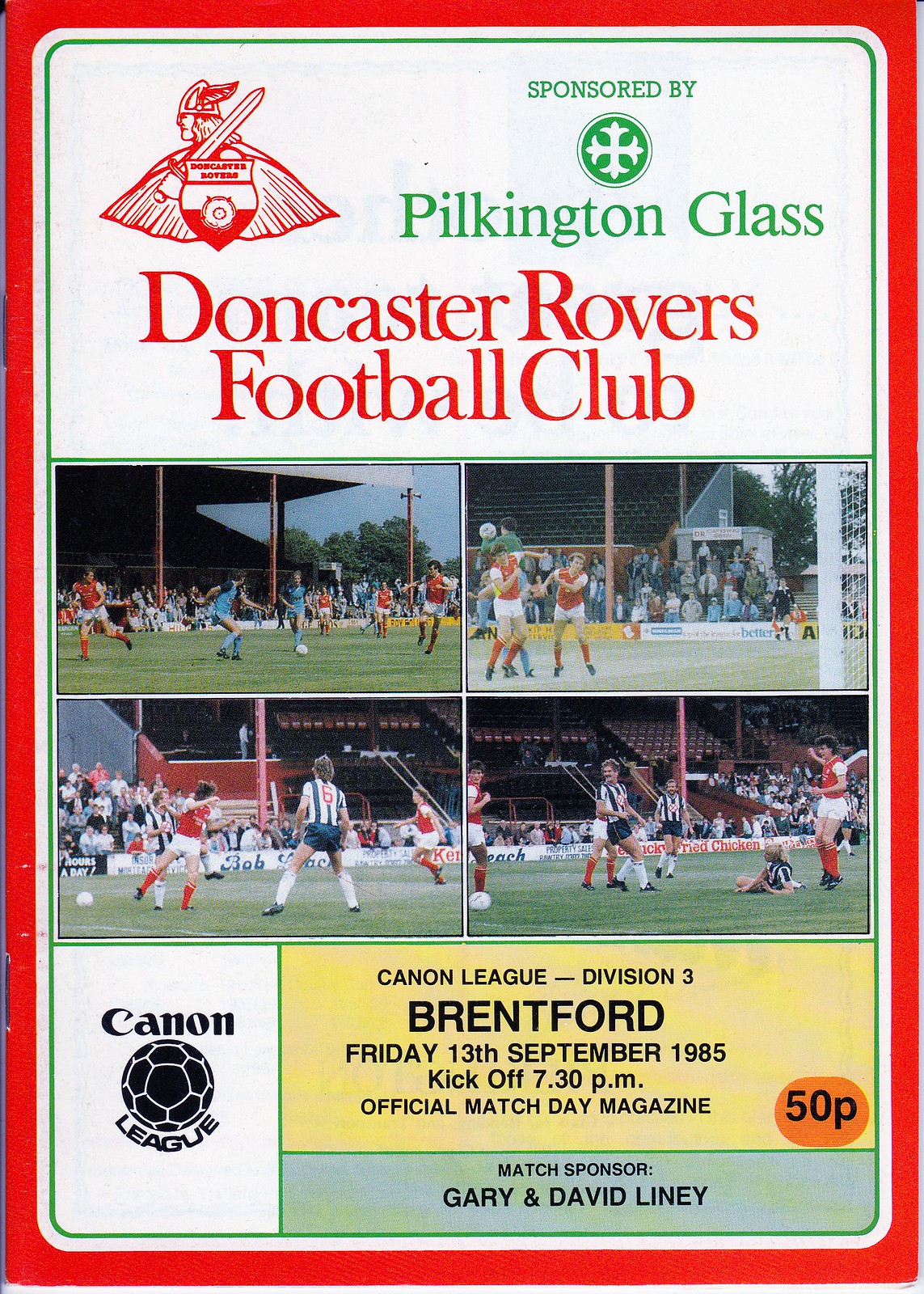The front cover of the Doncaster Rovers Football Club match day program features a clean white background bordered by a red frame. At the top, the text "Sponsored by Pilkington Glass" is prominently displayed in green. Centered on the left side is the red Doncaster Rovers logo, accompanied by the club’s name. Below the logo are four color photographs capturing dynamic soccer action on a green, grassy field with spectators in the stands. The bottom section includes a detailed match listing: a white rectangle with the "Canon League" logo and a soccer ball, followed by a yellow rectangle with black text announcing "Canon League Division 3, Brentford, Friday, 13th September 1985, kickoff 7.30 p.m., official match day magazine 50p." The match is sponsored by Gary and David Linney.